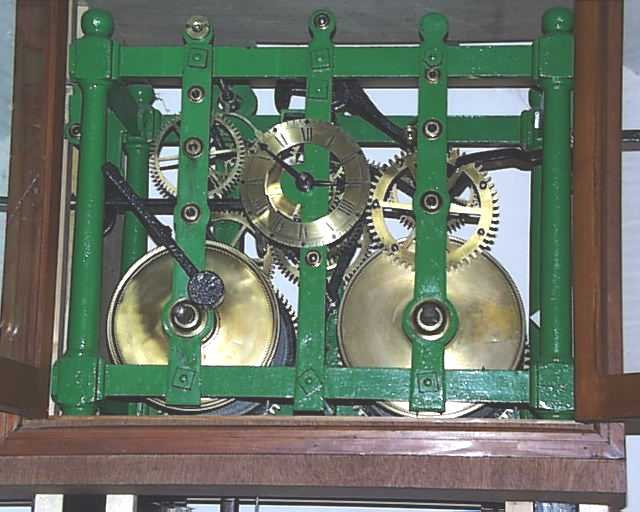This color photograph captures the intricate rear view of a clock, focusing on its internal mechanisms. Within the clock, there are about five bronze gears arranged in a circular pattern, integral to the timekeeping function. These gears are housed within a green-painted metal cage, which seems both sturdy and meticulously crafted. Surrounding this green metal structure is a broader wooden frame, giving the entire piece a classic, almost antique appearance. The inner mechanism also features a small central circle with Roman numerals and black hands, encased in gold, which stands out amidst the gears. The backdrop is a mix of dark brown wood and a lighter, possibly white, background, which adds depth and contrast to the overall image. Though it is somewhat ambiguous whether the wooden elements form part of the clock’s design or the environment it is placed within, the rectangular framing suggests it is housed within a wooden container or sitting on a wooden shelf.